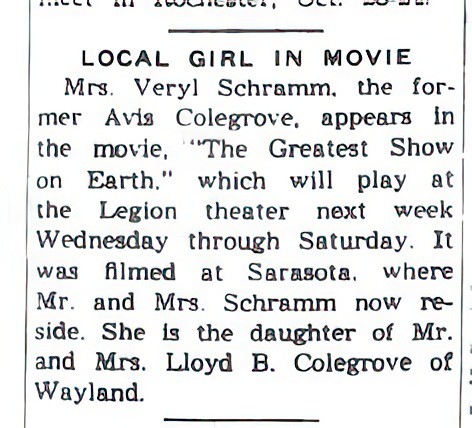The image is an excerpt from a vintage magazine advertisement featuring a solid white background with thin black font. The text reads, "LOCAL GIRL IN MOVIE," in all caps as a prominent headline. Below this, it continues, "Mrs. Verrill Shram, the former Avis Colgrove, appears in the movie 'The Greatest Show on Earth,' which will play at the Legion Theatre next week, Wednesday through Saturday. It was filmed at Sarasota, where Mr. and Mrs. Shram now reside. She is the daughter of Mr. and Mrs. Lloyd B. Colgrove of Wayland." Centered lines appear at the very top and bottom of the excerpt, with additional long lines running along both the left and right sides, framing the text in a classic newspaper advertisement style.